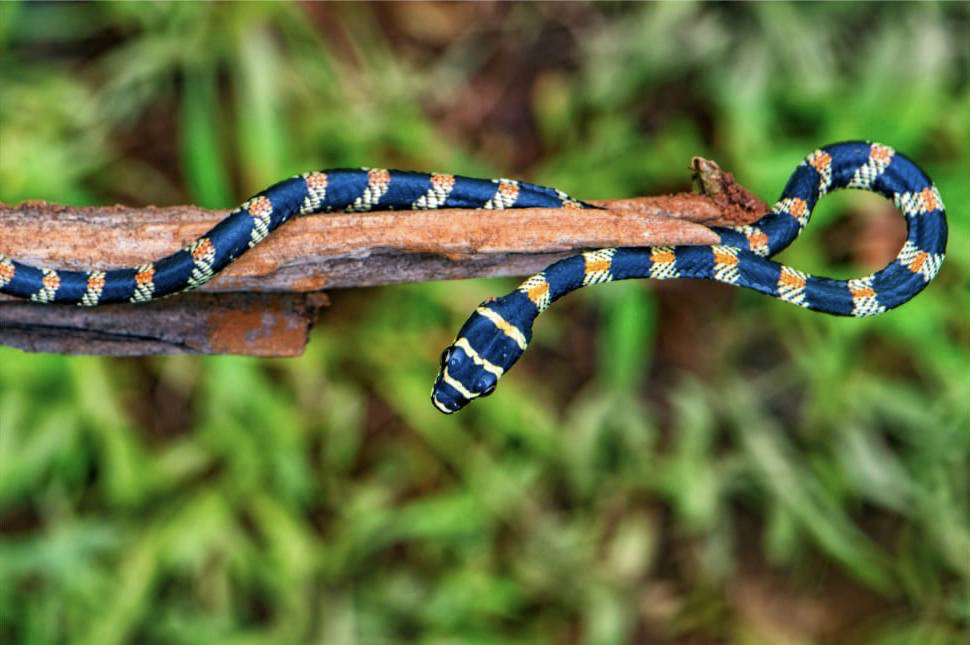This image showcases a vivid and slender snake, likely a corn snake, elegantly draped on a piece of wood that stretches from the left to the right edge of the frame before looping back towards the center. The snake, displaying a striking alternating color pattern, features thick black segments interspersed with yellow portions adorned with a prominent orange stripe running continuously along its body. Its head, positioned centrally in the composition, is marked by distinctive yellow stripes. Though the background is blurred, it hints at a lush, green forest floor, enhancing the vibrant contrast of the snake's brilliant colors. The wood, possibly a branch with a rusty-orange hue, further accentuates the vividness of the scene. The snake’s black eyes and overall slender, elongated form add to the detailed intricacy of this bright, vibrant photograph.